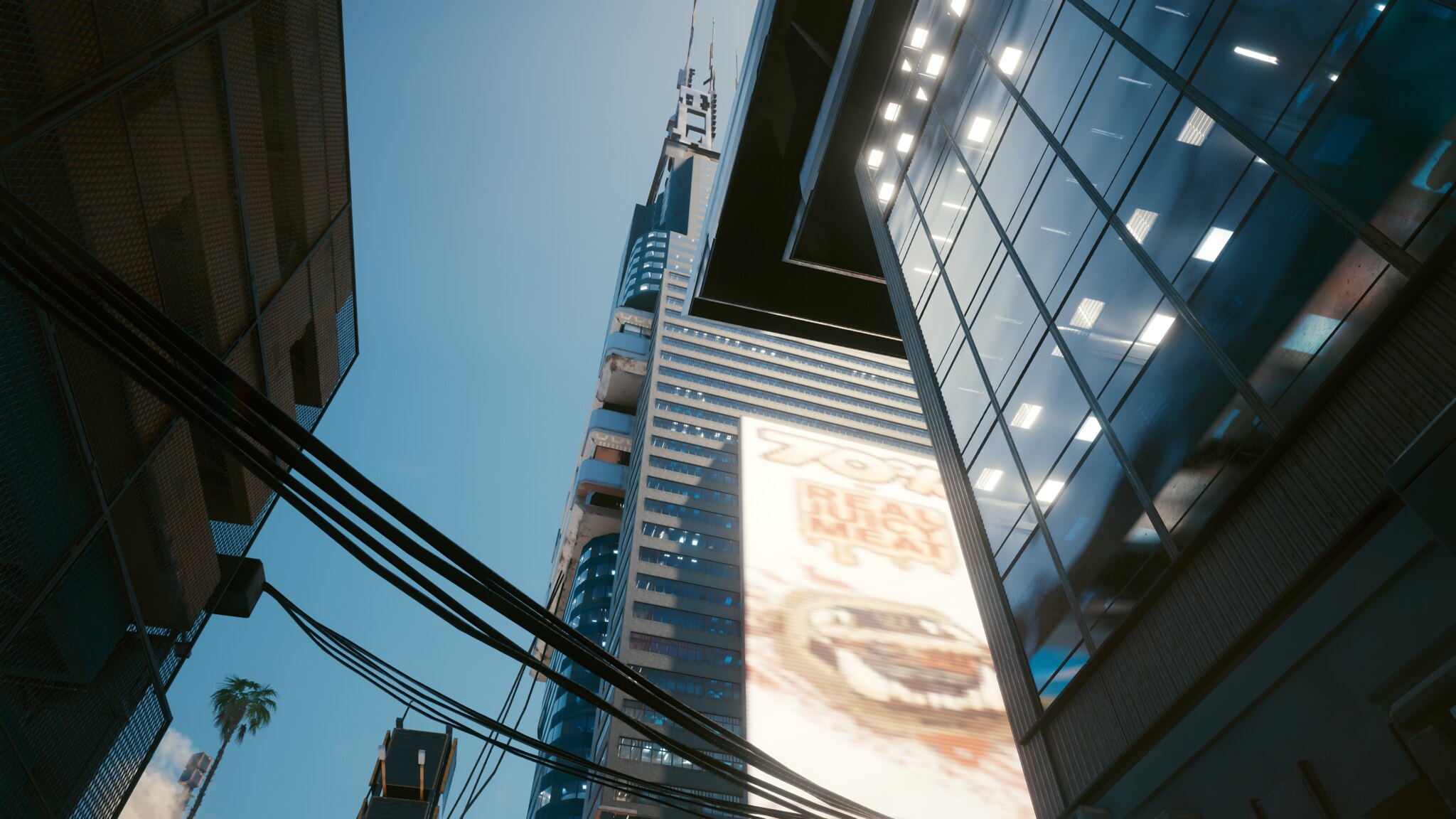A person stands in a bustling downtown area, gazing upward and capturing a photograph of towering buildings. The image prominently features the side of a colossal building that stretches all the way to the top, adorned with various antennas and other equipment. In the lower left corner, power lines are seen extending across the road, linking one building to another. The structure directly in front of the photographer showcases an extensive white billboard, emblazoned with a cartoonish dog with oversized, gleaming canine teeth and comically exaggerated eyes. Above the illustrated dog, the billboard proclaims "Real Juicy Meat," with a partially legible brand name noted above the text. This advertisement, promoting dog food, is affixed to a tall building peppered with numerous windows. At the very summit of this edifice, additional antennas are conspicuously mounted.